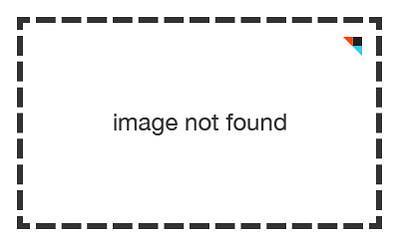The image depicts a white rectangular shape bordered by black dotted lines. In the center of the rectangle, there is black text that reads "image not found," with all letters in lowercase. Inside the top right corner of the rectangle, just within the dashed border, there's a small right-angled triangle. The triangle is divided into three sections: a black square on its top right side, a light blue section along the bottom, and a dark orange section on the left.